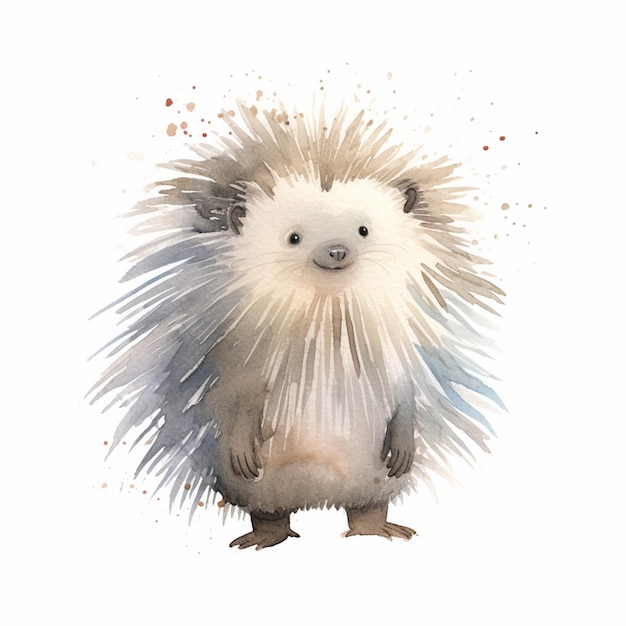This is a detailed illustration, likely a watercolor, depicting a cute hedgehog standing on its hind legs. The hedgehog is positioned slightly turned to the right but faces directly forward with a charming smile and black eyes. The fur is a soft blend of colors: brown on the top of its head and around its eyes, white on its face, and a mix of grayish-blue, brown, and gray on its arms and legs. Its paws are facing downward, and cute ears peek through the fur. In the background, there are splotches of brown and light brown paint, creating a halo effect around the head. The soft and professional rendering gives the image a soothing, almost ethereal quality.